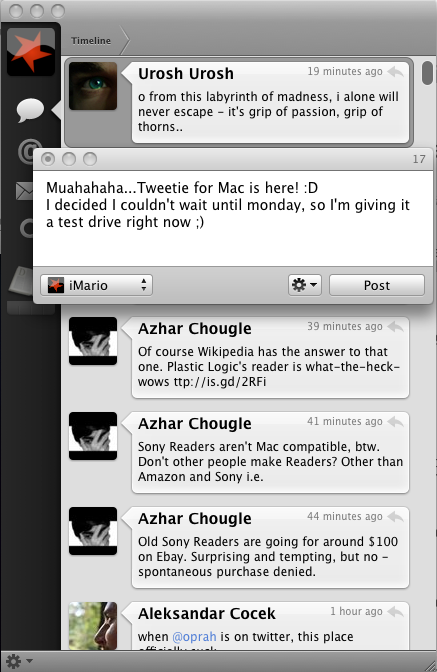The image is a detailed screenshot, possibly from a smartphone, showcasing a series of text or instant messages on a gray metallic background. Along the left side, there is a vertical column featuring several icons. The bottom of the image is bordered by a similar gray-silver strip with another icon on its left side. The main content displays six messages arranged in a vertical column. The top message is from a user named "Yurosh Yurosh" who posted 19 minutes ago: "Oh, from this labyrinth of madness, I alone will never escape its grip of passion, grip of thorns." Below it, a user named "iMario" has a message about to be posted, saying: "Mwahahahaha. Tweety for Mac is here. I decided I couldn't wait until Monday, so I'm giving it a test drive right now." Subsequent messages are from "Azhar Chougle," discussing e-readers: one mentioning that Wikipedia provides answers, another about Sony readers not being Mac compatible, and a third noting old Sony readers' prices on eBay. The final message, partially cut off, is from "Alexander Kosek," which starts: "When @Oprah is on Twitter this place..."